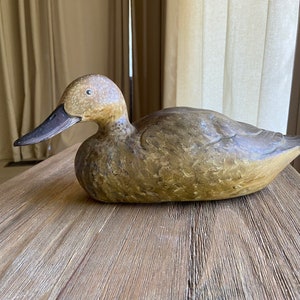In this detailed image, we see a meticulously crafted wooden sculpture of a mallard duck sitting on a clean, wooden table that features distinct lines. The mallard has a striking orange head paired with a light tan face, accentuating its black beak, and a darker, robust body. Its eyes are prominently visible, adding to the realistic detail of the piece. Situated against a backdrop of a white and a brown curtain, the scene is well-lit but doesn't specify whether taken indoors or outdoors, or the time of day. The photo, seemingly taken from a standing or kneeling position, offers a clear side view of the mallard, which is facing left. The absence of text in the image allows all focus to remain on the lifelike sculpted mallard, enhancing its visual impact.